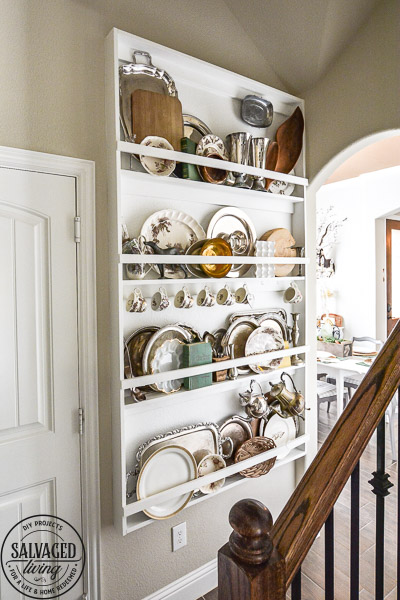In this detailed photograph taken inside a home, the focus is on a prominent and somewhat awkwardly placed large white shelving unit. Positioned at the corner of a hallway, near the front door and kitchen, this unit seems to dominate the wall space, emphasizing its significant size and storage capacity. The shelves, totaling four in number, are filled with an assortment of items including plates, cutting boards, trays, mugs, teapots, charger plates, and various trinkets. Noteworthy items on the shelves include a teal-colored book, a thin silver pan with scroll designs, a white plate with a gold rim, a black dog figurine, and a wooden cutting board at the top.

To the left of this imposing shelving unit, there is a white wooden door, and on the top right of the image, an arched doorway without a doorframe reveals a glimpse into an adjacent living room. The corner where the shelf is positioned features walls in a beige-to-white gradient, contributing to a well-lit and inviting atmosphere. On the bottom right of the photograph, a wooden staircase with a black railing can be seen leading upwards. Adding a unique touch, the bottom left corner of the image includes a small black stamp that reads "Salvaged Living." The overall scene captures a mix of practical storage and decorative elements within a cozy and lived-in home environment.